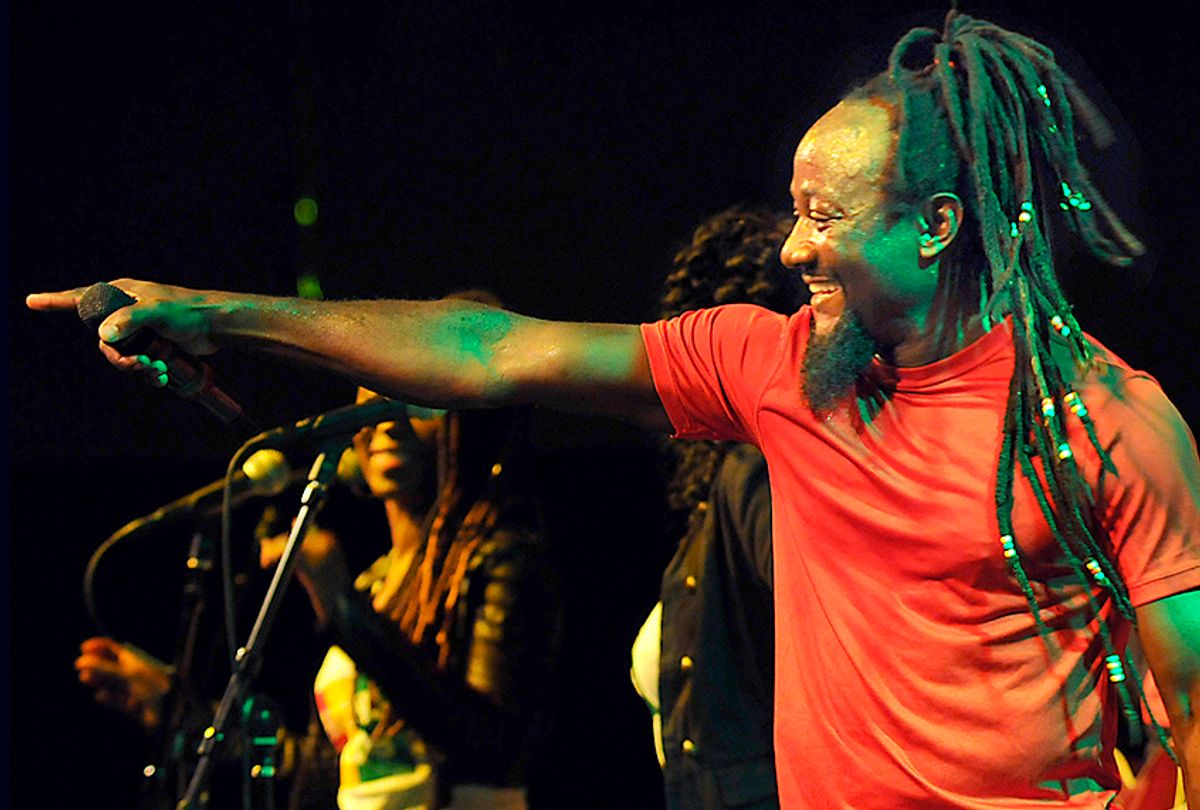In this vibrant image, we see a dynamic performance featuring a charismatic male singer prominently in the foreground. He is captured from a side view, sporting a bright red, slightly wrinkled t-shirt that contrasts strikingly with his dark skin tone. His face, adorned with a broad, joyous smile and a black beard, is partially turned towards what seems to be an audience. His long dreadlocks, embellished with green and white beads, sway with the energy of his movements. The singer's right arm is extended, his hand holding a black microphone while his pointer finger gesticulates towards someone off-frame to his right.

In the background, partially obscured by the man's expressive pose, stand two female performers. One, positioned near the center of the composition, is barely visible except for glimpses of brown, curly hair and her attire featuring a black shirt over a white undershirt. The other, more to the left, has striking orange hair and is caught in a moment of mirth, smiling broadly while dressed in a white t-shirt. Both women have microphones in front of them, hinting at their roles in the performance.

The scene is enveloped in a deep black backdrop, lending a stark contrast that keeps the focus firmly on the performers while creating an atmosphere brimming with the potential of a captivating live show.